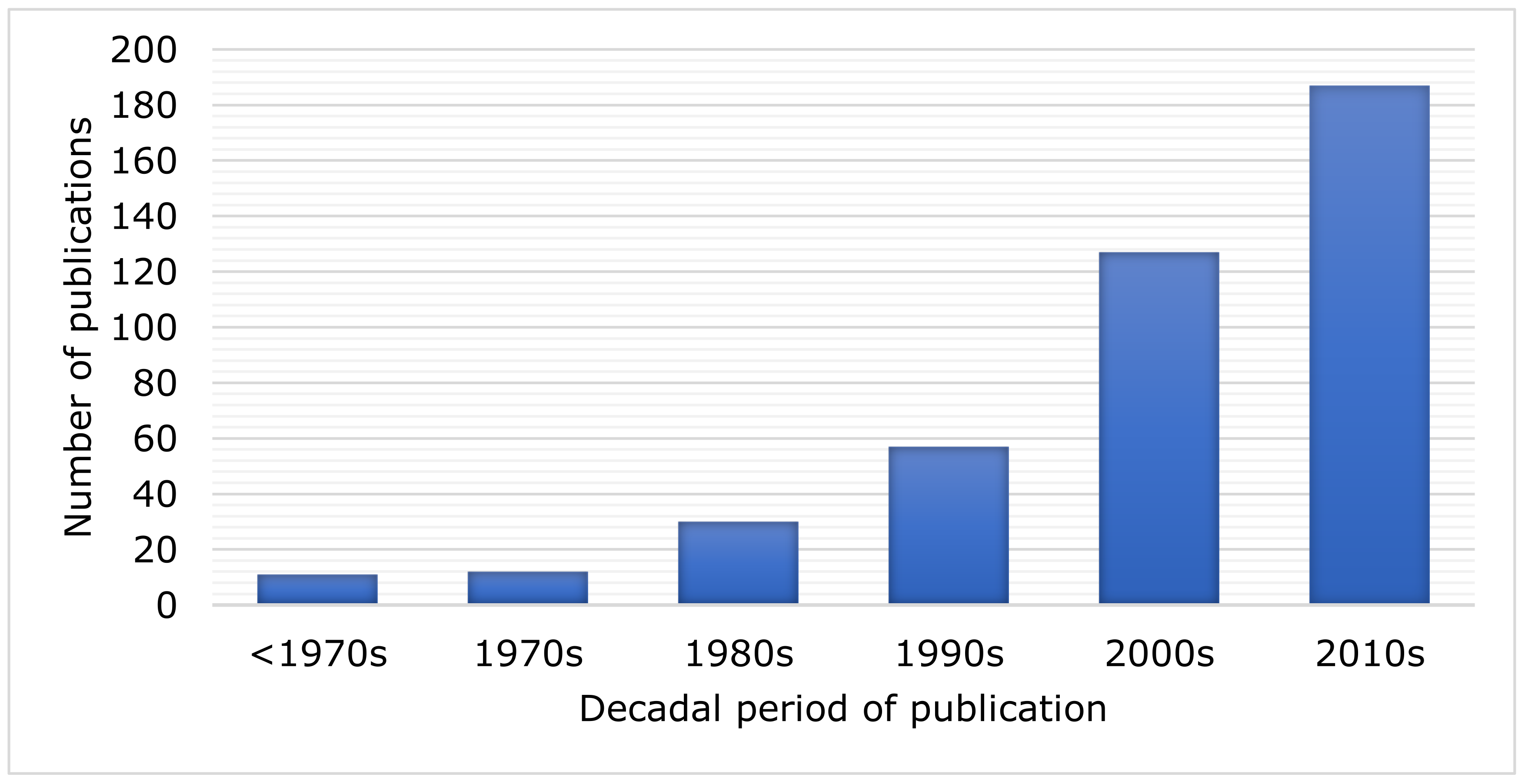The image features a detailed bar graph illustrating the number of publications per decade. The Y-axis, labeled "Number of Publications," ranges from 0 to 200 in increments of 20. The X-axis, labeled "Decadal Period of Publication," spans from "Before 1970s" to the "2010s." The bars, filled in with an opaque dark blue, indicate a significant growth in publications over time. Initially, the count remains modest, with less than 20 publications before the 1970s. The numbers then begin to double approximately each decade, from around 10-12 in the 1970s to about 185 by the 2010s. This substantial increase highlights a dramatic rise in the number of publications over the surveyed decades. The graph, predominantly black and white except for the blue bars, succinctly captures the exponential growth in scholarly output from the 1970s onwards.